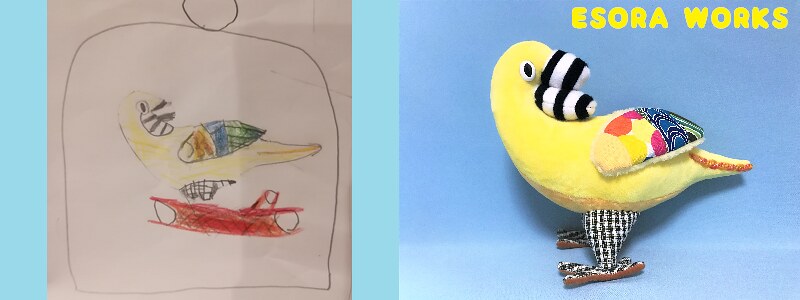The image is divided into two sections. On the left, there is a child's drawing on a sheet of white paper set against a light blue background. The drawing features a yellow bird with a colorful brown wing, plaid-looking legs, and a striped beak, standing on a red surface that resembles a child's snow sled. The bird is depicted looking over its shoulder. Above the drawing, the company name "Isora Works" is written in yellow text.

On the right side of the image, there is a photograph of a plush toy created based on the child's drawing. The toy bird is made of plush material and mirrors the drawing with its yellow body, colorful wings that sport a paisley design and orange, yellow, and pink circles, houndstooth-checkered legs, and striped beak. The toy stands on its feet. At the top right of this section, the company name "Isora Works" appears again in yellow text.

The entire image demonstrates a service where a child's drawing can be turned into a stuffed animal, illustrating the company's creative transformation from drawing to plush toy.